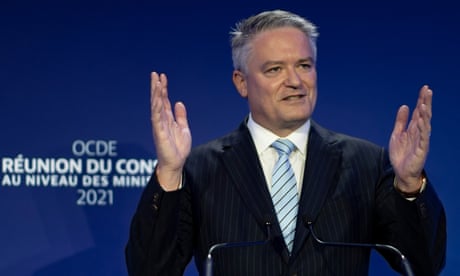In the image, a man appears to be giving a speech or presentation at a conference. He stands mid-frame, wearing a navy blue pinstripe suit, a white button-up shirt, and a light blue striped tie. His salt-and-pepper hair is neatly parted, and he is using both hands, raised to the sides, as if emphasizing a point. In front of him are two skinny black microphones positioned at chest height. The background is a dark blue screen with white text that reads "OCDE Reunion" and additional obstructed words in French, along with the year "2021." The man’s mouth is slightly open as he speaks, and his watch can be seen on his left wrist. The setting and attire suggest a formal event, likely involving a professional or academic presentation.